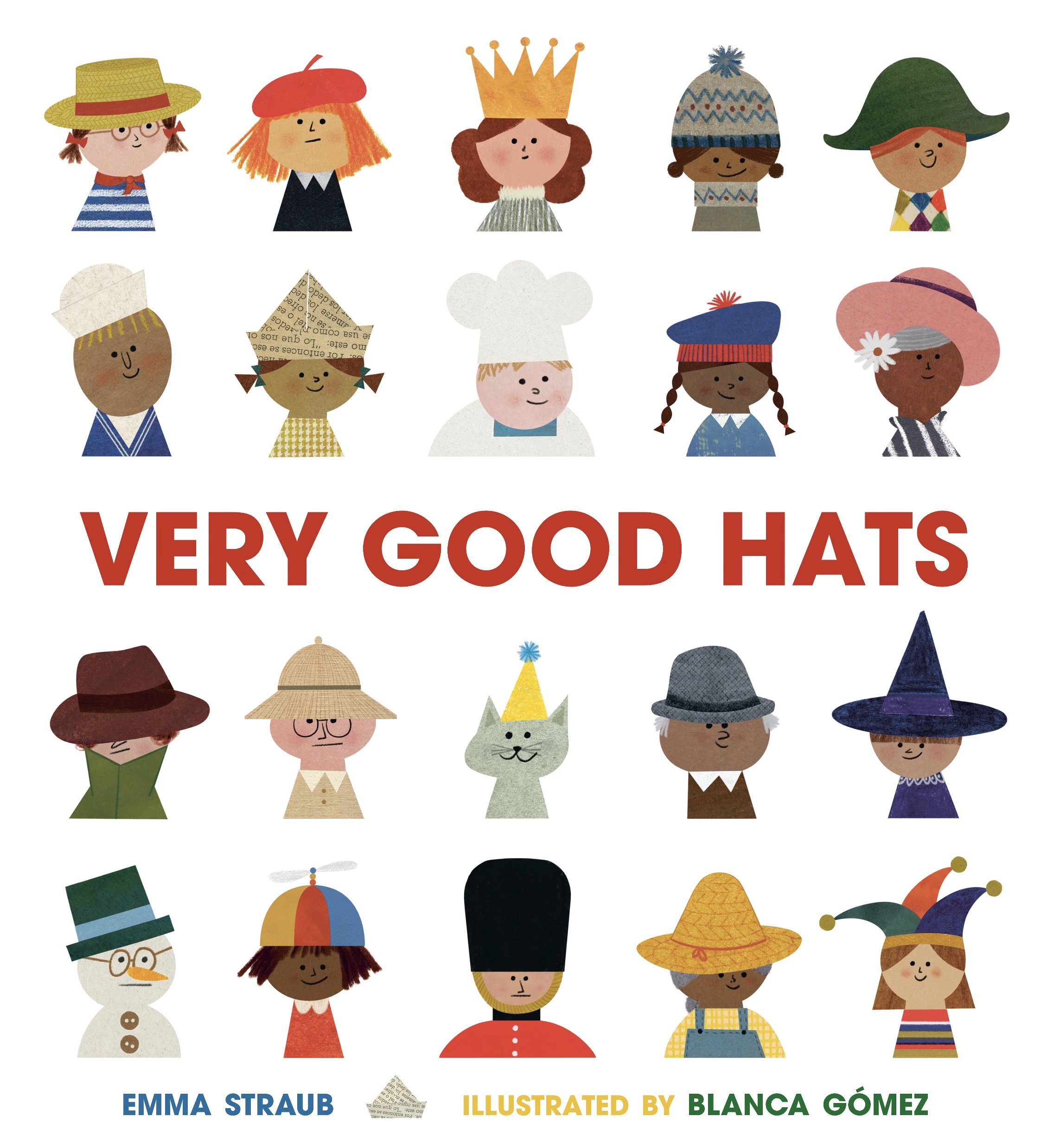The cover illustration of Emma Straub's children's book, "Very Good Hats," illustrated by Blanca Gomez, features a delightful array of twenty cartoon characters across four rows, all donning a variety of playful and culturally distinctive hats. From the top left, we see a little girl dressed as a gondolier complete with a red boater hat and striped blue shirt, followed by a girl with a French beret, another with a gold queen’s crown, a girl with a winter snow hat, and one with a Napoleon-style hat. The variety continues with characters sporting a sailor hat, a newspaper hat, a chef hat, a party hat, a detective hat, and an explorer hat. Not limited to humans, the collection also includes a cat in a hat, a figure in a bowler hat, a witch hat, a snowman in a hat, and an English guardsman’s hat. Each character, from a farmer to a jester and a cowboy, brings their unique charm, contributing to the overarching theme captured in the bold red lettering at the center declaring, "Very Good Hats." This vibrant assembly likely hints at an engaging and whimsical content that celebrates the diversity and fun of different hats and the stories they tell.